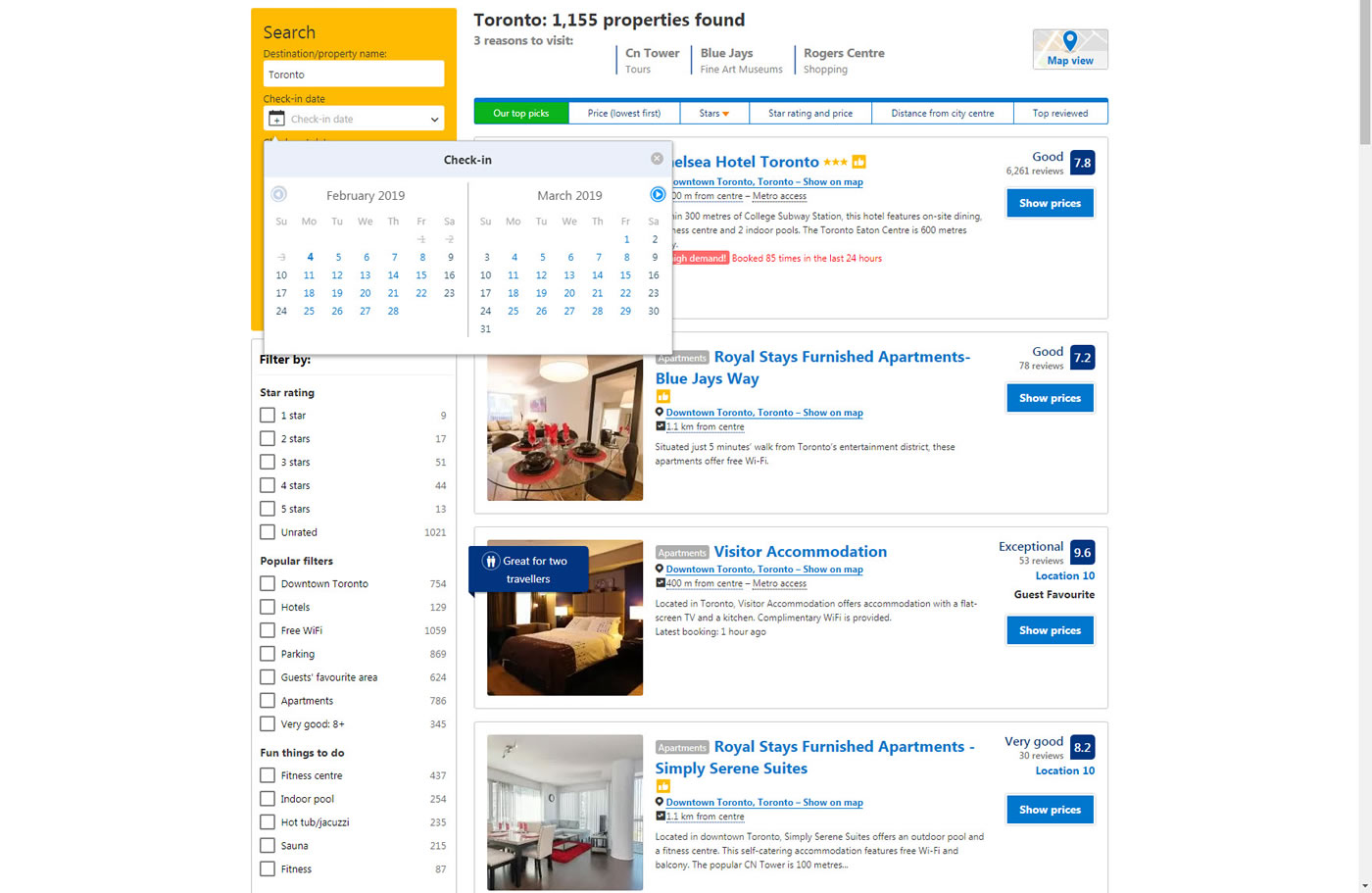**Caption:**

A comprehensive listing of 1,155 apartment properties in Toronto is prominently displayed, with an introduction at the top highlighting three main reasons to visit the city: CN Tower tours, Blue Jays games, fine art museums, and shopping at Rogers Centre. On the top right of the listing is an option for "Map View," and on the left, a yellow section labeled "Search" allows users to refine their query. This search bar features a white box for entering a destination or property name, preset with "Toronto." Below, there are fields for selecting check-in dates, separated into February 2019 and March 2019 calendars.

Further down, users can filter their search by star ratings, popular filters, and fun activities nearby. To the right of the page, four prominent listings are showcased: "Royal Stays Furnished Apartments on Blue Jays Way," "Visitor Accommodation," "Royal Stays of Furnished Apartments," and "Simply Serene Suites." Each listing includes a photo of the apartment on the left, a description, and a score indicating its rating.